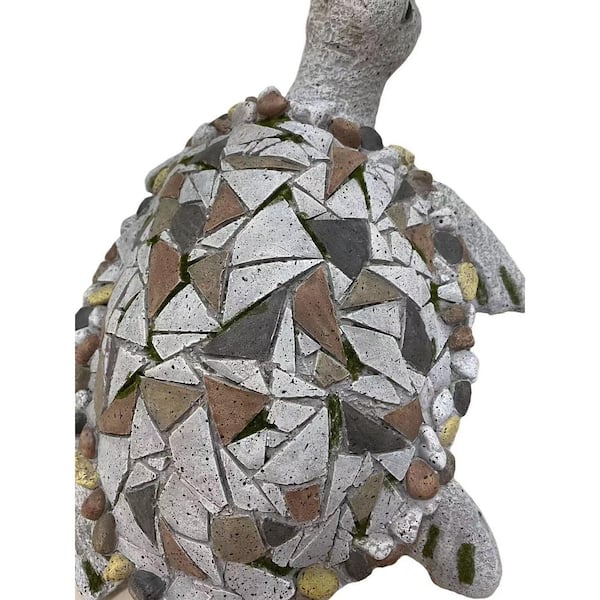The image depicts a photorealistic turtle sculpture, set against a plain white background. The turtle is not positioned head-on but oriented to the left, revealing its rightmost fin, front and back fins, and a partial view of its head with a drawn eye. The sculpture, primarily made of gray rock, features a detailed mosaic shell composed of various shard-like pieces. These pieces include different shades of gray, brown, and black, along with small brown and gold-colored rocks forming the shell's ornate edging. The elliptical shell's surface hosts both triangular and circular stones, giving it a textured appearance. Greenish-gray markings on the fins add further texture to the sculpture. The entire piece, suggestive of a garden sculpture, exhibits intricate craftsmanship and a harmonious blend of natural hues.